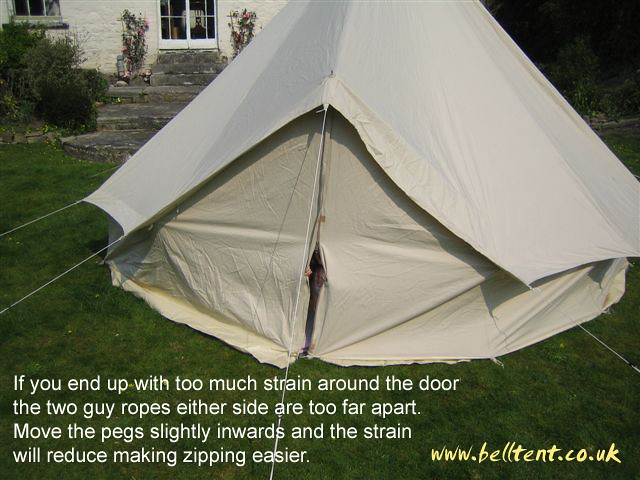This is a detailed color photograph of a white canvas tent, resembling a teepee or yurt, set up on a lawn that appears to be the backyard of a house. The tent, with a zippered front entry, is positioned near the center of the image. In the background to the left, there are stone steps and a white doorway of a house, featuring white brick walls and surrounded by some flowers and shrubbery. The image contains clear instructions in white text at the bottom left corner, which reads, "If you end up with too much strain around the door, the two guy ropes on either side are too far apart. Move the pegs slightly inwards and the strain will reduce making zipping easier." Additionally, the bottom right corner displays an advertisement in yellow text, "www.belltent.co.uk." The tent's front opening is slightly ajar, showing a hand unzipping it from inside.